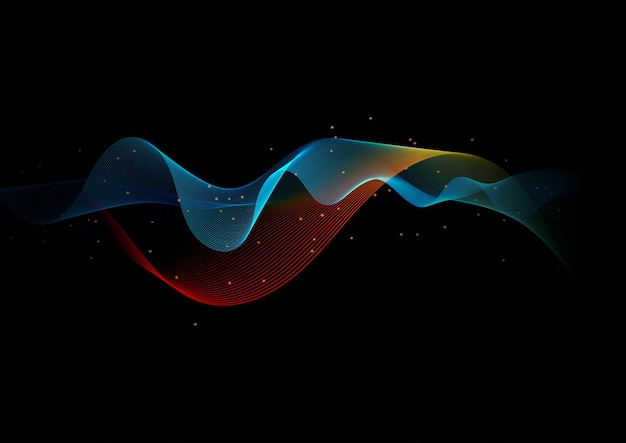This digital art image presents an evocative scene of two intertwining waves set against a black background reminiscent of a cosmic night sky. The blue wave, which undulates irregularly like a sound wave, traverses horizontally across the frame. Below it is a red wave that mirrors the sound wave form, displaying ribbed internal lines. As these translucent waves overlap and interconnect in places, they blend into vibrant hues of yellow and touches of green, adding depth and dynamic color shifts. Scattered throughout the background are numerous tiny yellow dots that evoke the twinkle of distant stars, enhancing the surreal and ethereal quality of the image. This powerful visual composition is akin to the abstract cover art of Pink Floyd's "The Dark Side of the Moon," with both waves and background working together to create a mesmerizing, otherworldly atmosphere.